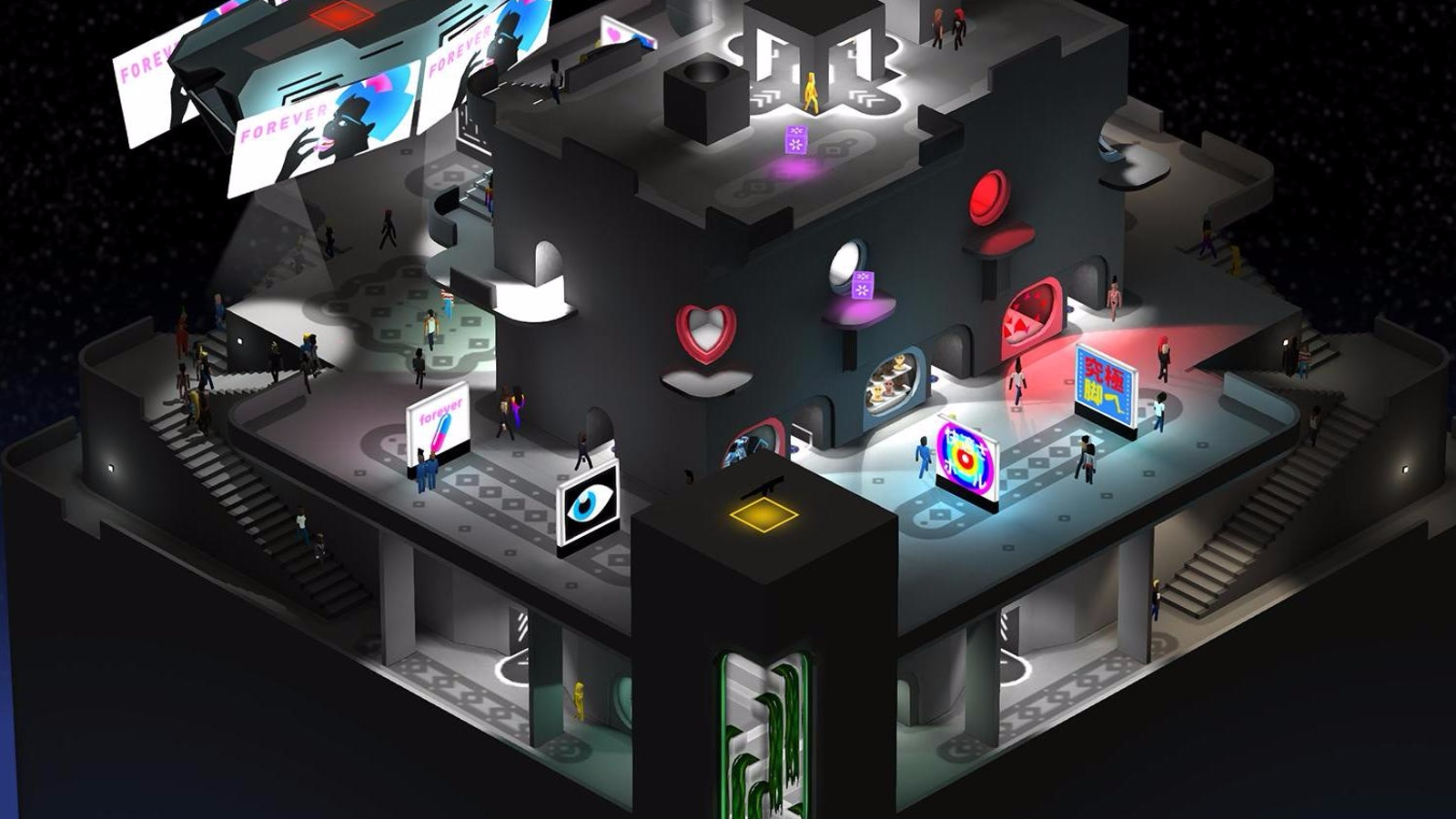The image features a 3D model of a futuristic city, set against a stark black background. The cityscape is turned towards the viewer in a diamond-shaped orientation, offering a corner view of its multi-level structure. The model spans three distinct stories, with black and gray being the dominant hues. Splashes of color highlight billboards, signs, and kiosks throughout the structure, providing a stark contrast to the otherwise monochromatic theme. 

On the left-hand side, a set of MC Escher-like gray stairs ascends from the first to the second level, populated by small human figures adorned in various clothing and hair colors, contributing to the scene's bustling ambiance. The first level features numerous cube-like structures with indentations that might serve as rooms or housing units, each identified by a symbol and a color such as a red heart or a lavender light.

Prominent on the top left are two distinctive, brightly colored billboards. One displays the word "forever" in pink and depicts a monster consuming a pill. Another sign features foreign characters and vibrant hues including red, yellow, and blue. Scattered elsewhere are more signs inscribed with the word "forever," one of which shows an eye with blue elements.

The much smaller top level, or the third level, houses an illuminated central cube accessible from all sides, though its purpose remains enigmatic. The overall atmosphere of the model suggests a fantastical, open-air urban environment, somewhat resembling a sprawling, surreal mall. This imaginative and intricate representation of a futuristic city captivates with its detailed and visually engaging elements.